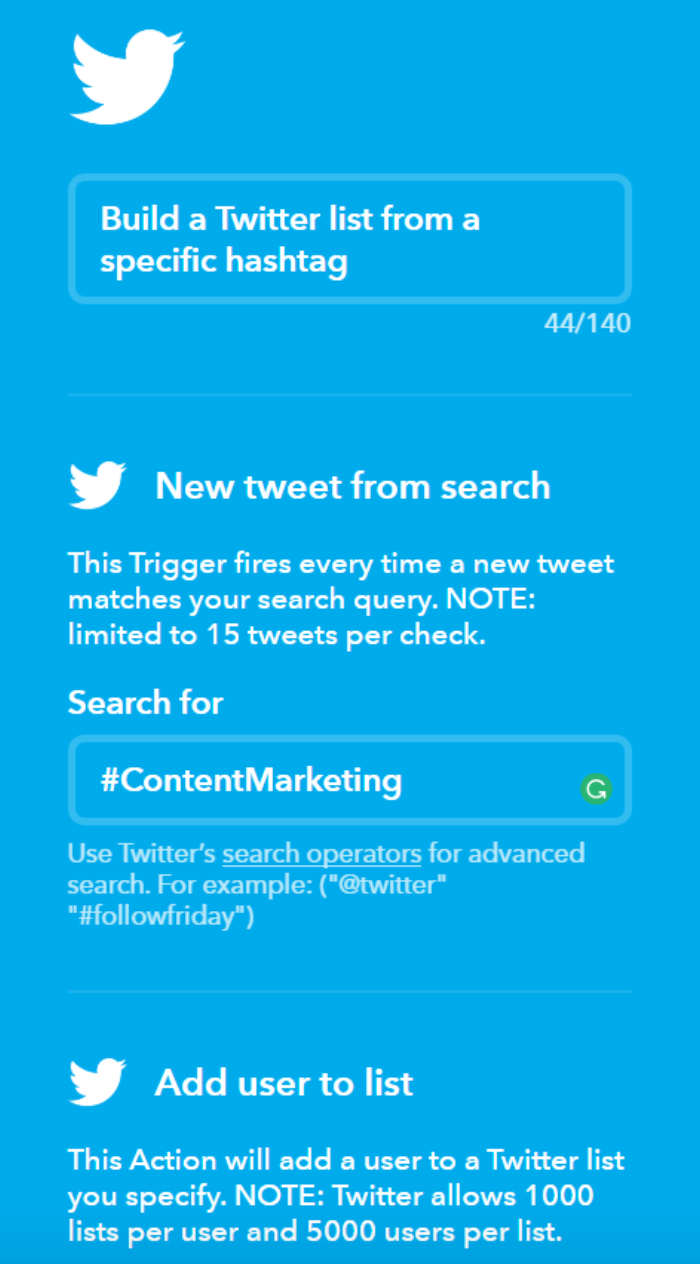In this vertically oriented image, the classic Twitter logo is prominently featured against a sky-blue background reminiscent of the original Twitter iconography. In the upper left corner, there's a white Twitter bird icon angled upwards, flying to the right. Alongside it, the text reads: "Build a Twitter list from a specific hashtag. 44 of 140 characters used." 

Below this, another Twitter bird icon introduces a section that states, "New tweet from search. This trigger fires every time a new tweet matches your search query. Note: Limited to 15 tweets per check. Search for #contentmarketing with a refresh. Use Twitter's search operators for advanced search (e.g., @Twitter and #FollowFriday)." 

Further down, the bird logo appears once more, followed by the instructions: "Add user to list. This action will add a user to a Twitter list you specify. Note: Twitter allows 1,000 lists per user and 5,000 users per list."

The image is detailed and informative, focusing on utilizing Twitter's functionalities for list building and advanced tweet searches.